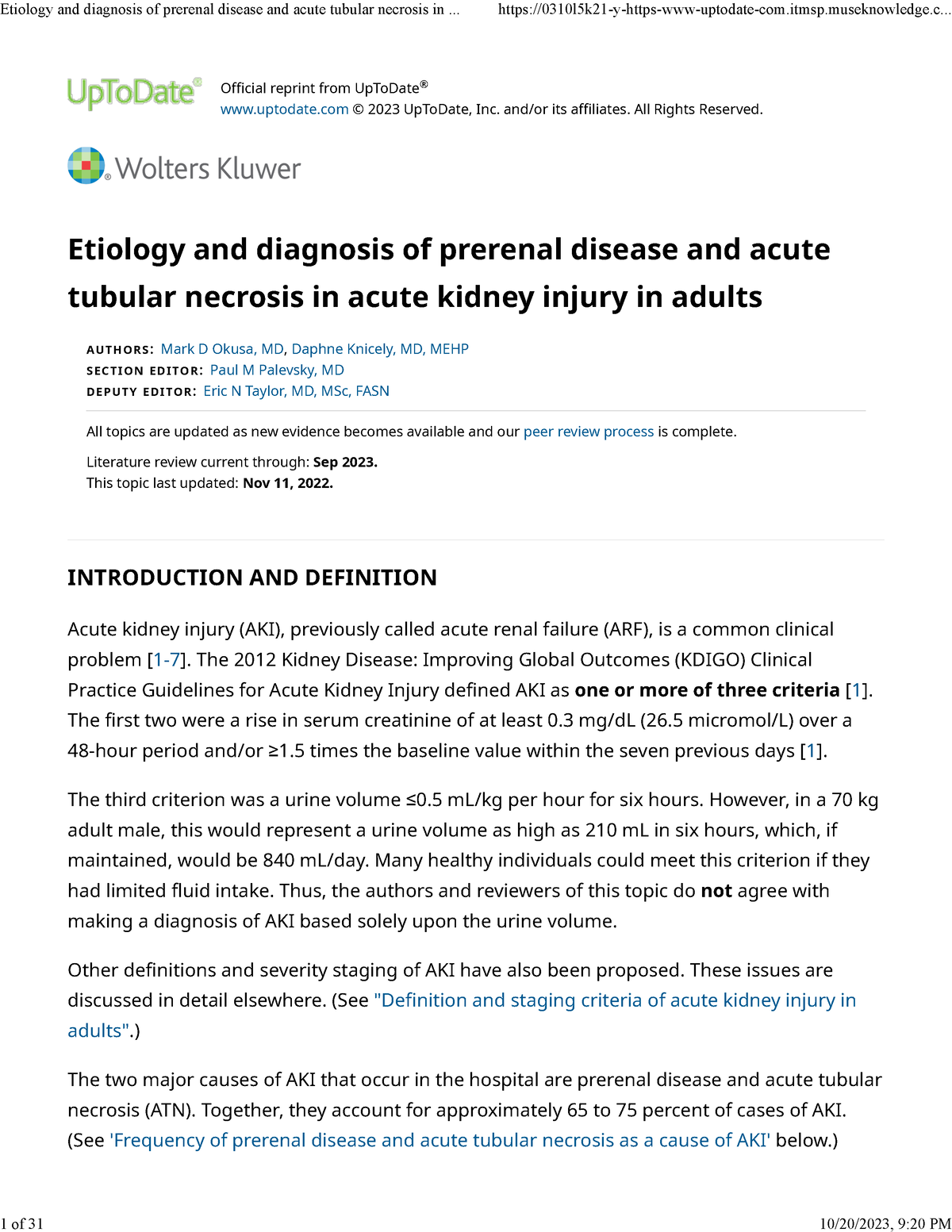**Descriptive Caption:**

This image depicts a webpage from the UpToDate medical resource platform. The webpage features a clean, white background with text presented primarily in a standard, professional font. In the upper left-hand corner is a small-text header with what appears to be a non-black font color, making the text somewhat difficult to read. The visible text includes terms related to the "Ecology and Diagnosis of Perineal Disease," "Acute Tubular Necrosis," and "Acute Kidney Injury in Adults." To the right of this header, a website link is displayed.

Directly below this section, the webpage specifies that the content is an "official reprint from UpToDate." The statement is followed by the webpage's URL, "uptodate.com," along with the copyright details: "2003 UpToDate, Inc. and/or its affiliates. All rights reserved." Adjacent to this text is the logo for "Wolters Kluwer," with the logo icon situated to the left of the company name.

The title of the article, prominently displayed, is "Ecology and Diagnosis of Perineal Disease and Acute Tubular Necrosis and Acute Kidney Injury in Adults." Below the title, the webpage lists the names of the authors, the section editor, and the deputy editor. The literature review is noted to be current through September 2023, with the latest update made on November 11, 2022. The webpage then transitions into the main content, beginning with sections labeled "Introduction and Definition," followed by several detailed paragraphs explaining the subject matter of the article.